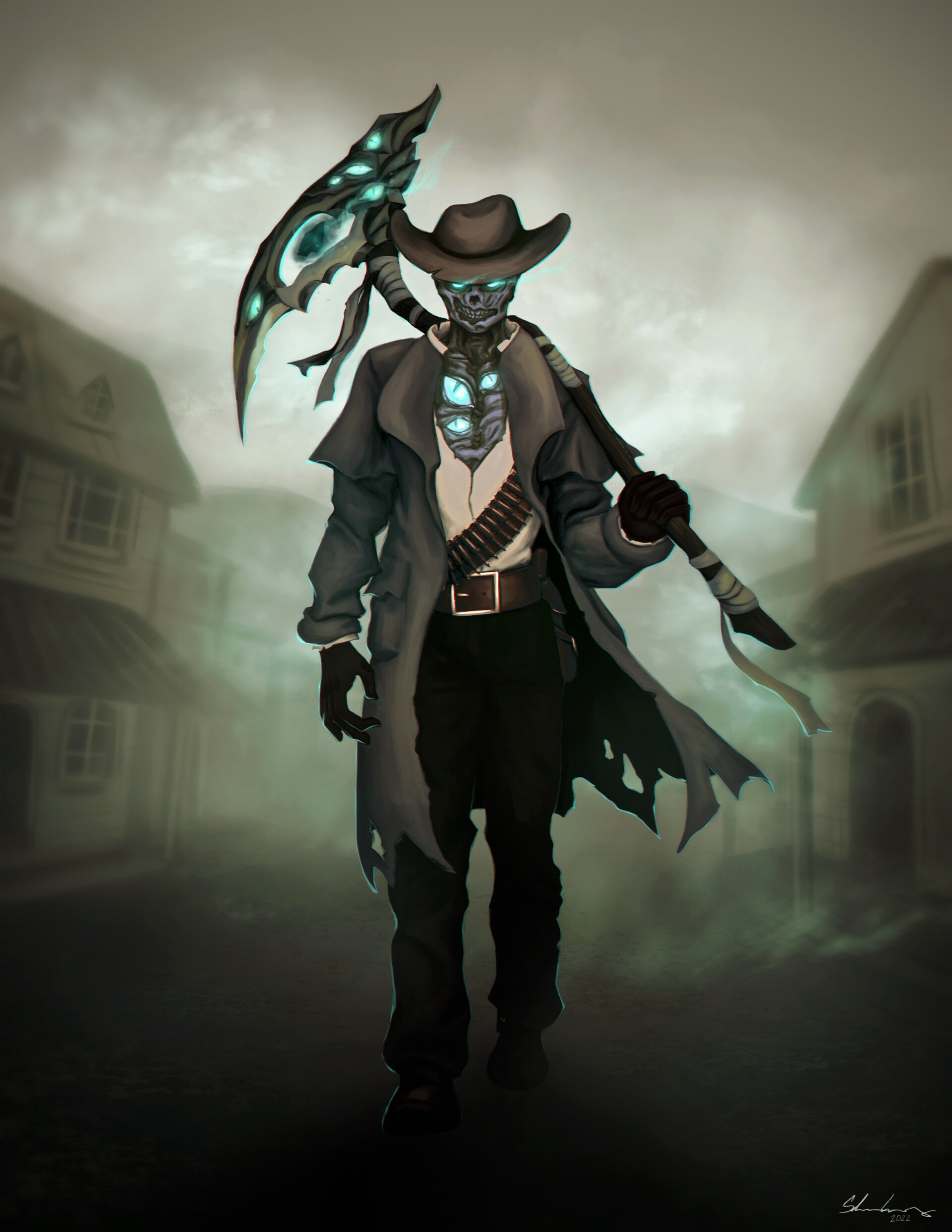This image is a detailed cartoon drawing set in a portrait layout, in which the top and bottom are shorter than the sides. It features a menacing, cowboy-like skeleton walking through a foggy and murky town. The signature in the lower right corner is unintelligible and is written in white, with the date "2022" beneath it. The background is dark and smoky, partially obscuring the buildings on either side of the character, creating an eerie atmosphere.

The skeleton, positioned prominently in the center, is donned in elaborate attire: a tall cowboy hat, a long brown tattered coat, black gloves, black pants, a brown belt with a gold buckle, and boots. He wears a beige or white vest that reveals part of his chest. The chest area, along with his eyes, emits a teal blue or green glow.

He is armed with a sickle held in his left hand and has ammunition strapped across his chest. Additionally, he appears to have some sort of winged or wide tie-like accessory with blue sections. The character's skeletal grin and glowing eyes accentuate his menacing presence as he walks down the smoky, fog-laden street.